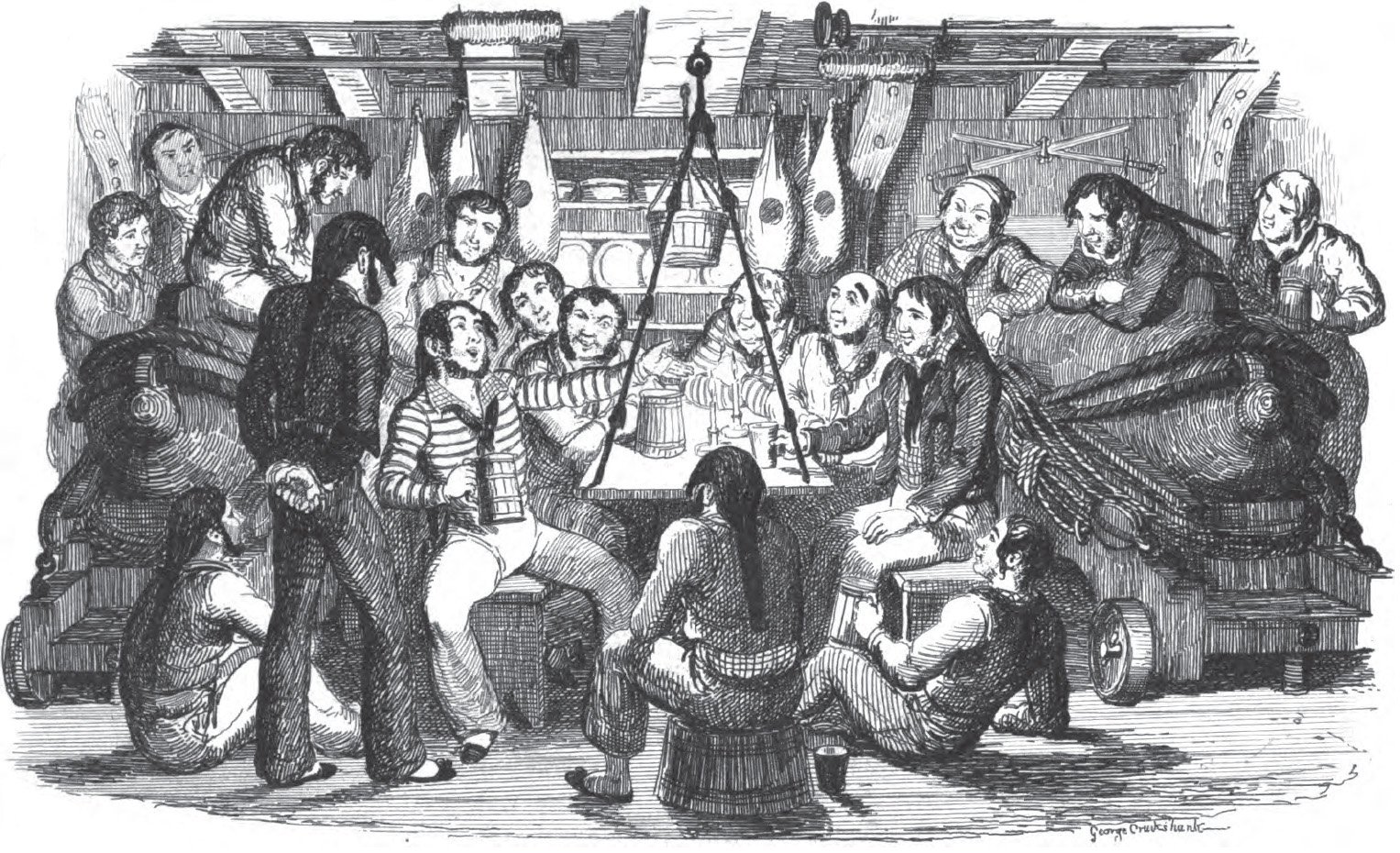In this detailed black and white pencil drawing, approximately twenty men are gathered in what appears to be the below-deck area of a sailboat, indicated by the wooden floors and ceiling. A table, suspended from ropes, forms the central focus, adorned with drinks and candles. The scene is lively, with crew members dressed in striped long-sleeve shirts, black ties, and white pants, loosely gathered around the table. Among them is one man with long black hair tied in a ponytail, who is animatedly telling a story, beer mug in hand, as his shipmates attentively listen. The atmosphere suggests camaraderie and casual conversation, further accentuated by the presence of two men propped up against what appear to be cannons, contributing to the nautical setting.